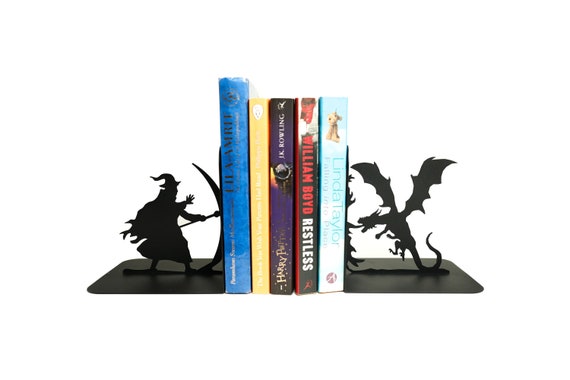This image showcases an elegant display of four books held upright by two unique, intricately-designed bookends. On the left side, the bookend takes the shape of a wizard clad in a long robe and characteristically pointed hat, wielding a staff that emanates a magical force forming an almost shield-like aura. His other hand is outstretched with fingers splayed, as if casting a powerful spell. This wizard closely resembles a character from the Wizard of Oz.

On the right side, the bookend features a majestic dragon in mid-flight, with its tail just touching the ground. The dragon, depicted in an all-black silhouette, is captured in a fierce pose with its mouth wide open, breathing fire towards the books. The detailed design highlights its expansive wingspan and menacing stance.

Between these fantastical bookends, four books stand tall. While the titles of the first two books from the left are unreadable, the third book is unmistakably a Harry Potter novel by J.K. Rowling. The fourth book is "Restless" by William Boyd, and the last book, authored by Linda Taylor, has an unreadable title. This carefully arranged display captures the viewer's attention with its mystical and literary charm.